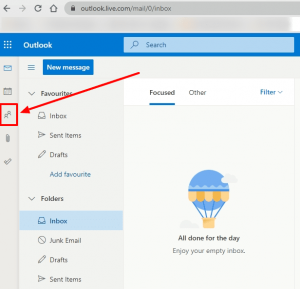The image displays a detailed interface of the Outlook email platform. At the top of the screen is a gray informational search bar with the text "Outlook.live.com/mail/inbox" accompanied by a blue rectangle. Inside this rectangle, to the left, is the word "Outlook," and to the right, there is an elongated blue search bar featuring a magnifying glass icon on the left side. Directly beneath this search bar, located within a blue rectangle, is the text "New Message." 

A red arrow descends from the search bar and points diagonally to the left, leading to another area marked by a red square that contains two small gray dots, representing users. Behind this highlighted section, a sidebar lists several sections: "Favorites," which includes items such as "Inbox," "Sent Items," "Drafts," and "Add Favorite." Below this, under "Folders," are listed additional items: "Inbox" (highlighted in a blue rectangle), "Junk Email," "Drafts," and "Sent Items."

To the right of this sidebar, there is an image of a vibrant hot air balloon, primarily blue with yellow and orange accents. Below this image, the text reads "All Done for the Day," and further down in gray text, it says "Enjoy Your Empty Inbox." At the very top of this section, the word "Focused" is underlined in blue, indicating the current inbox view.